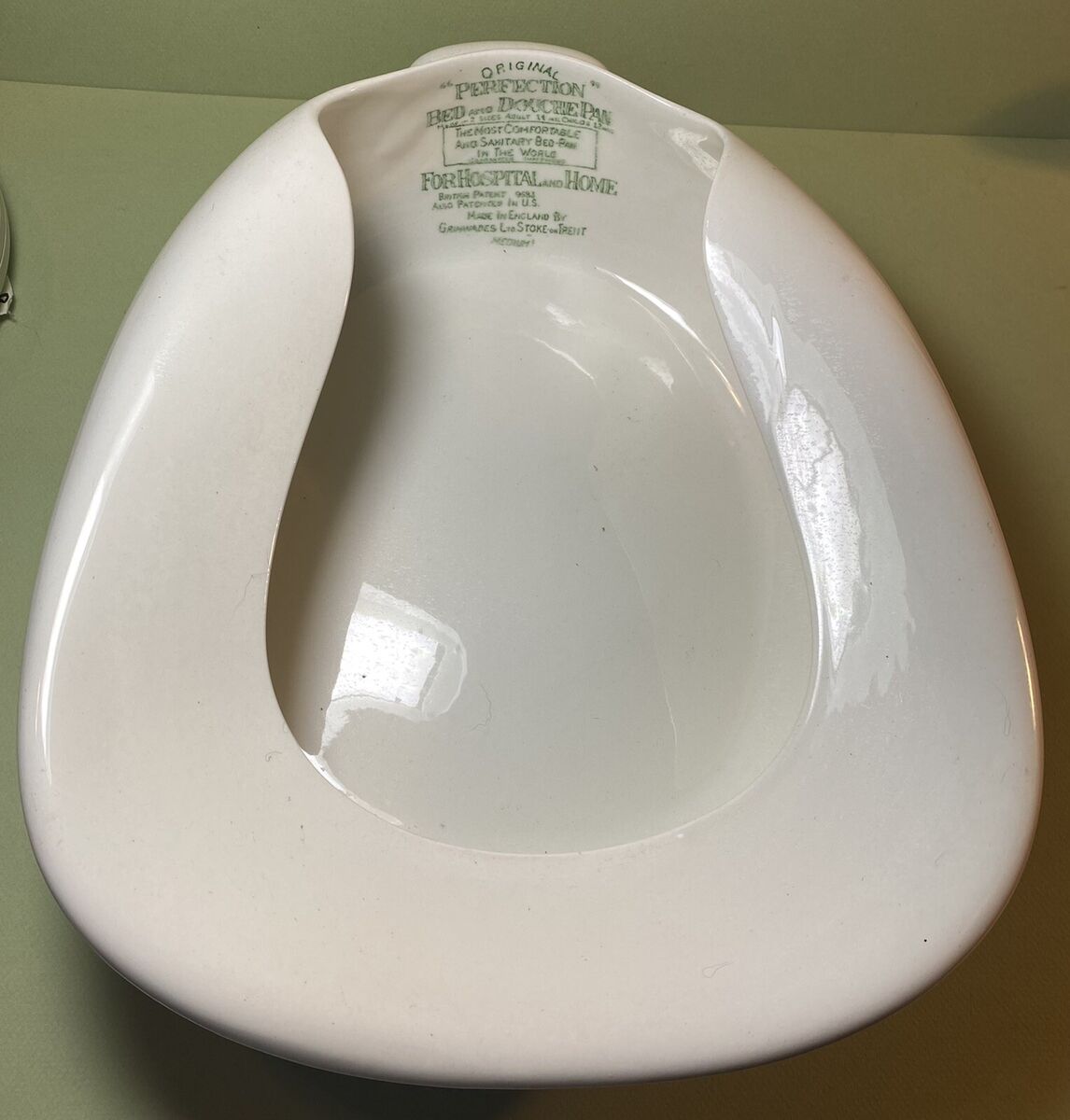The image showcases a white bedpan set against a green background. The bedpan appears somewhat reflective, suggesting it could be made of porcelain or plastic. Prominent, readable text at the top of the bedpan states "Original Perfection Bed and Douche Pan," which is marketed as "the most comfortable and sanitary bedpan in the world," intended for hospital and home use. Though it appears to be shaped like a toilet seat, it has an enclosed bottom, indicating its function for individuals who are unable to use a standard restroom. Additional writing on the bedpan mentions it is patented in the U.S. and manufactured in England, though some details are difficult to discern due to small text size. The item is described as medium-sized in blue lettering. Reflective lighting on the surface of the bedpan indicates the environment around it.